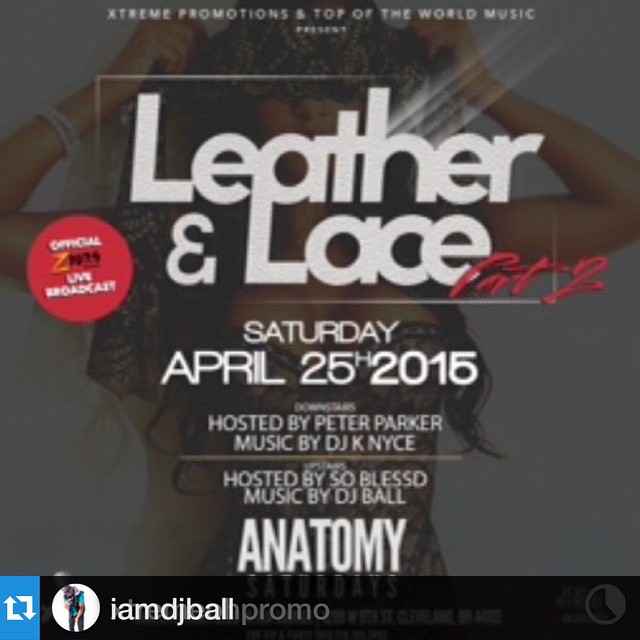The advertisement features a promotional image set against a grey background dominated by a large white headline reading "Leather and Lace." The central figure in the image is a woman dressed in black lingerie with her hands in her dark hair. Overlaid text announces "Extreme Promotions and Top of the World Music" present an event on "Saturday, April 25th, 2015." Despite some fuzziness, the flyer also mentions the event will be hosted by Peter Parker with music by DJ K. Nice NYC and DJ Ball. At the very bottom of the ad, the word "Anatomy" appears in large white letters against a black band, indicating the nightclub venue in Cleveland, Ohio. A smaller inset image of a woman alongside the white text "I am DJ Ball" and the grey text "Promo" is also visible. This flyer seems to be an announcement for a recurring event, specifically for part two of the "Leather and Lace" series.